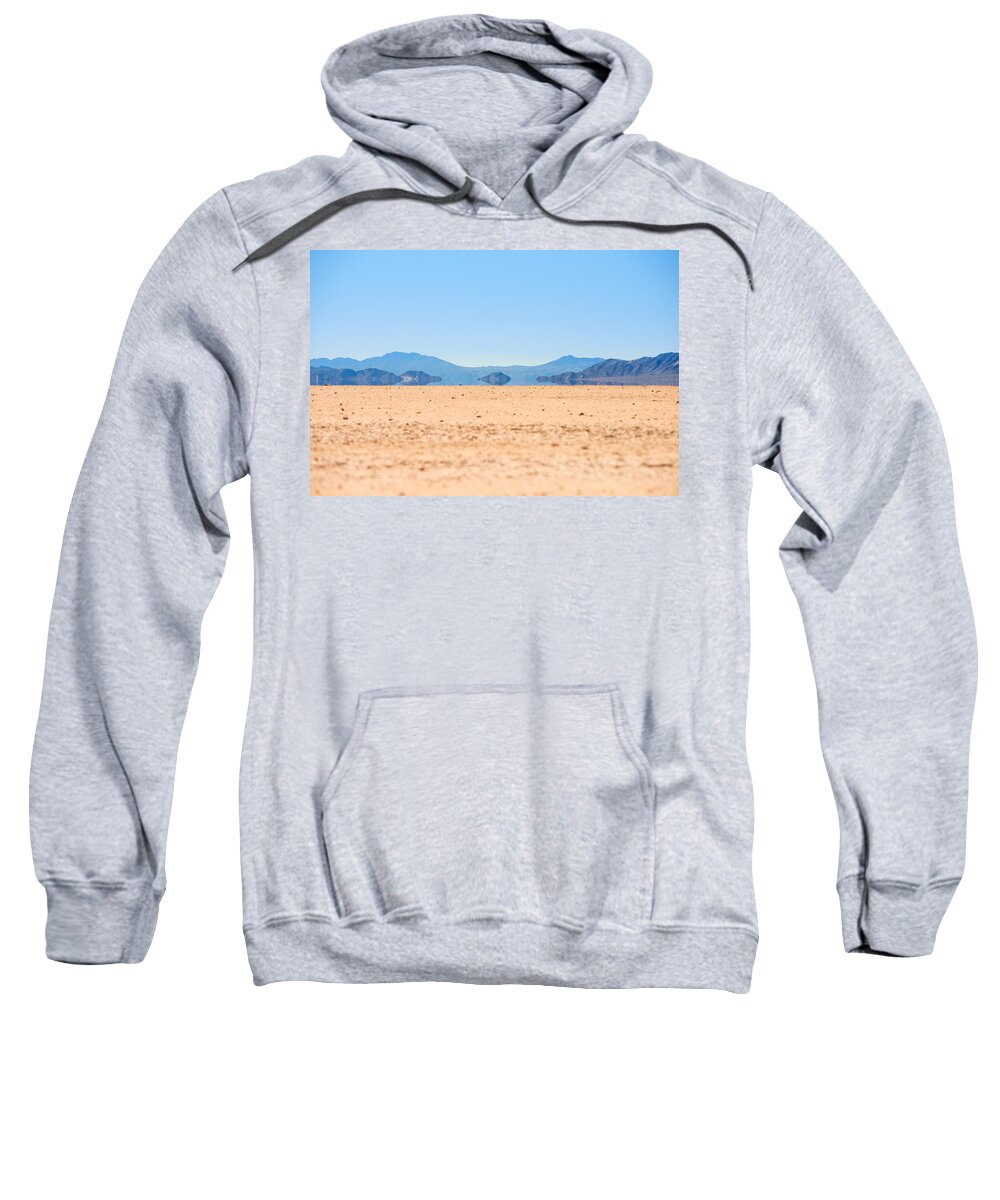This image depicts a light gray hooded sweatshirt set against a solid white background. The sweatshirt features darker gray or black drawstrings for the hood and a front pocket designed to accommodate both hands. At the center of the chest, there is a vibrant color photograph showcasing a barren desert landscape. The lower half of the photograph is dominated by light tan sands strewn with small rocks and pebbles. Rising from the sand, a distant range of brown and blue-tinged mountains extends across the image. The upper portion of the photograph captures a clear, bright blue sky with almost no cloud cover, amplifying the stark beauty of the desert scene. The image appears as if it has been printed onto the sweatshirt, emphasizing the arid and still atmosphere of a picturesque desert day.